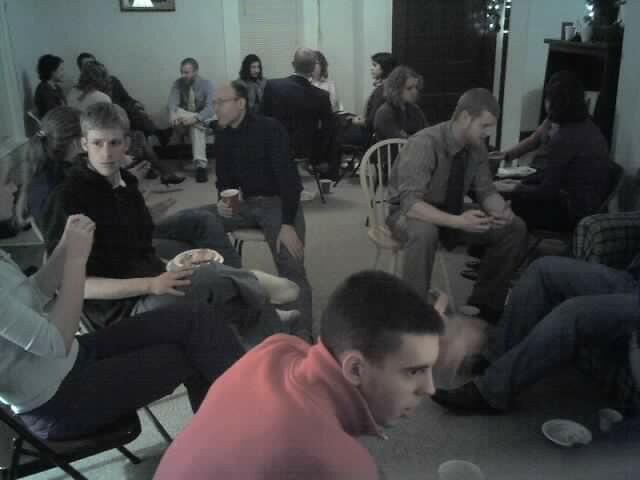The image depicts an indoor gathering in what appears to be either a hallway or a study room, characterized by a black, gray, and white background. A prominent individual in the foreground, a Caucasian man with short, dark hair shaved on the sides, is highlighted wearing a red polo shirt with the collar lifted up. He is holding a cup. The seating arrangement includes wooden and folding chairs, some placed in a circular formation, while others are arranged in no particular order, accommodating approximately 16 to 20 individuals.

The majority of attendees appear to be males in their late teens to early twenties, with a few older men displaying signs of balding. There is also a hint of a possible female presence, identified by a ponytail peeking out from behind one man. The overall setting suggests a casual social event, evident from a plate of food visible and several individuals holding cups. While most people are seated on chairs, some are on couches, contributing to the informal atmosphere of the gathering.